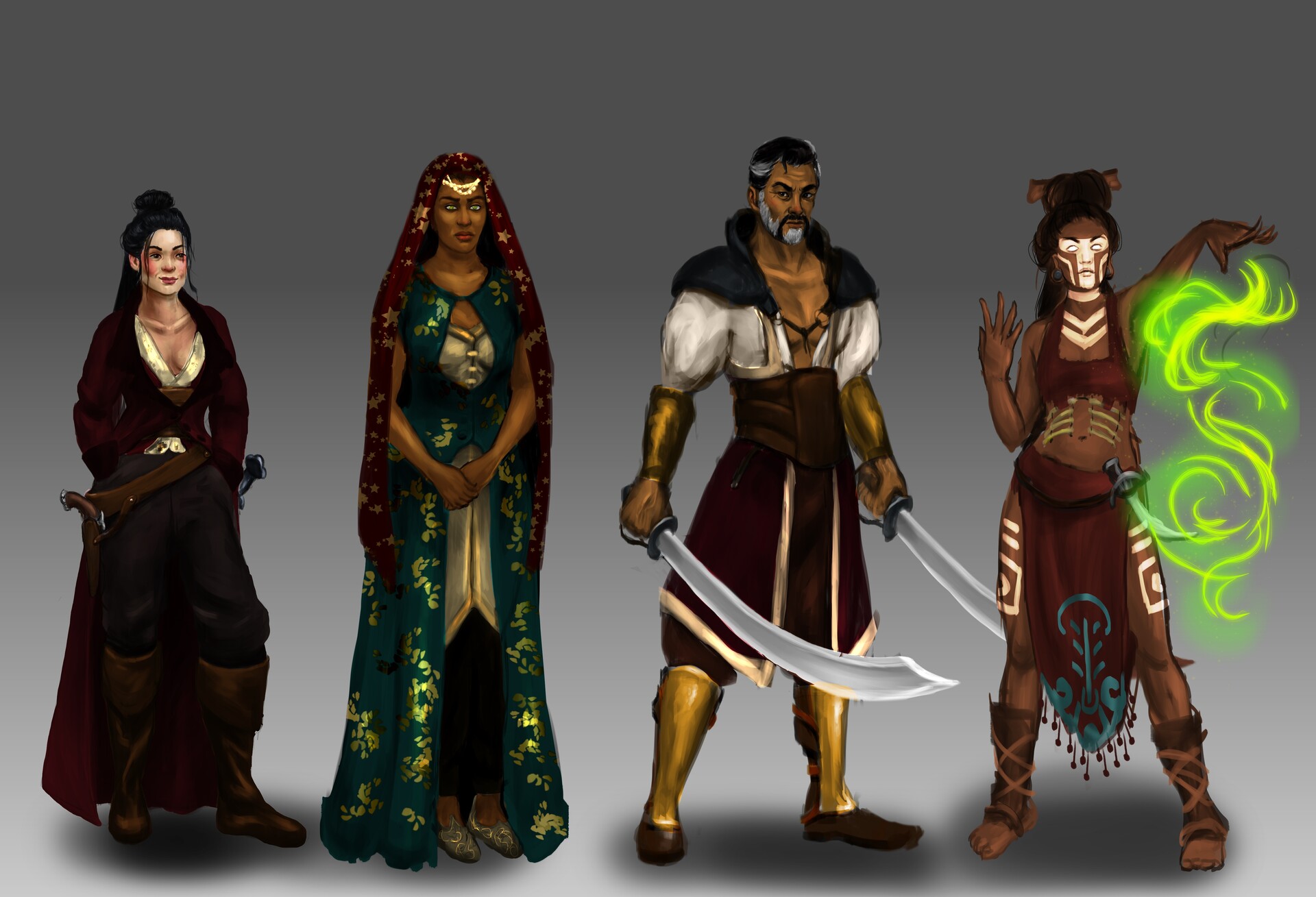This detailed illustration features four distinct fantasy characters standing in a row, evenly spaced from left to right, each exhibiting unique traits and vibrant colors. 

On the far left is a fair-skinned woman with black hair styled in a bun with a ponytail. She wears a long red coat over a white v-neck dress, complemented by black pants and tall brown leather boots. A brown belt with a holstered flintlock pistol and a sword on her hips accentuate her slightly pirate-like appearance.

Next, to her right, stands a woman adorned in a red and gold starry veil with glowing jewelry on her forehead. She wears a turquoise green button-up dress with silver-gold cloth around her chest and waist, paired with ankle-high slip-on shoes and black pants.

The third character is a man with a striking mix of gray and black hair and facial hair, featuring a goatee that is both black and white. He wears a white puffy shirt under black armor with gold shoulder pads and armbands on his forearms. His lower half is clad in a red Middle Eastern-inspired outfit with gold shin guards, and he wields two curved, silver Arabian-style swords.

Finally, the character on the far right is a mystical woman with her right hand raised, casting a spell with green neon swirls emanating from her palm. She has black hair in a bun adorned with a brown bone and her face is painted with white arrows, giving her a Native American aesthetic. She wears a red tank top revealing her belly and chest, a red loincloth, brown shin guards, boots, and sandals, all accentuated by white body paint.

The backdrop of this illustration is a neutral gray, highlighting the diverse and vibrantly colored fantasy characters, likely designed for a video game or similar entertainment medium.